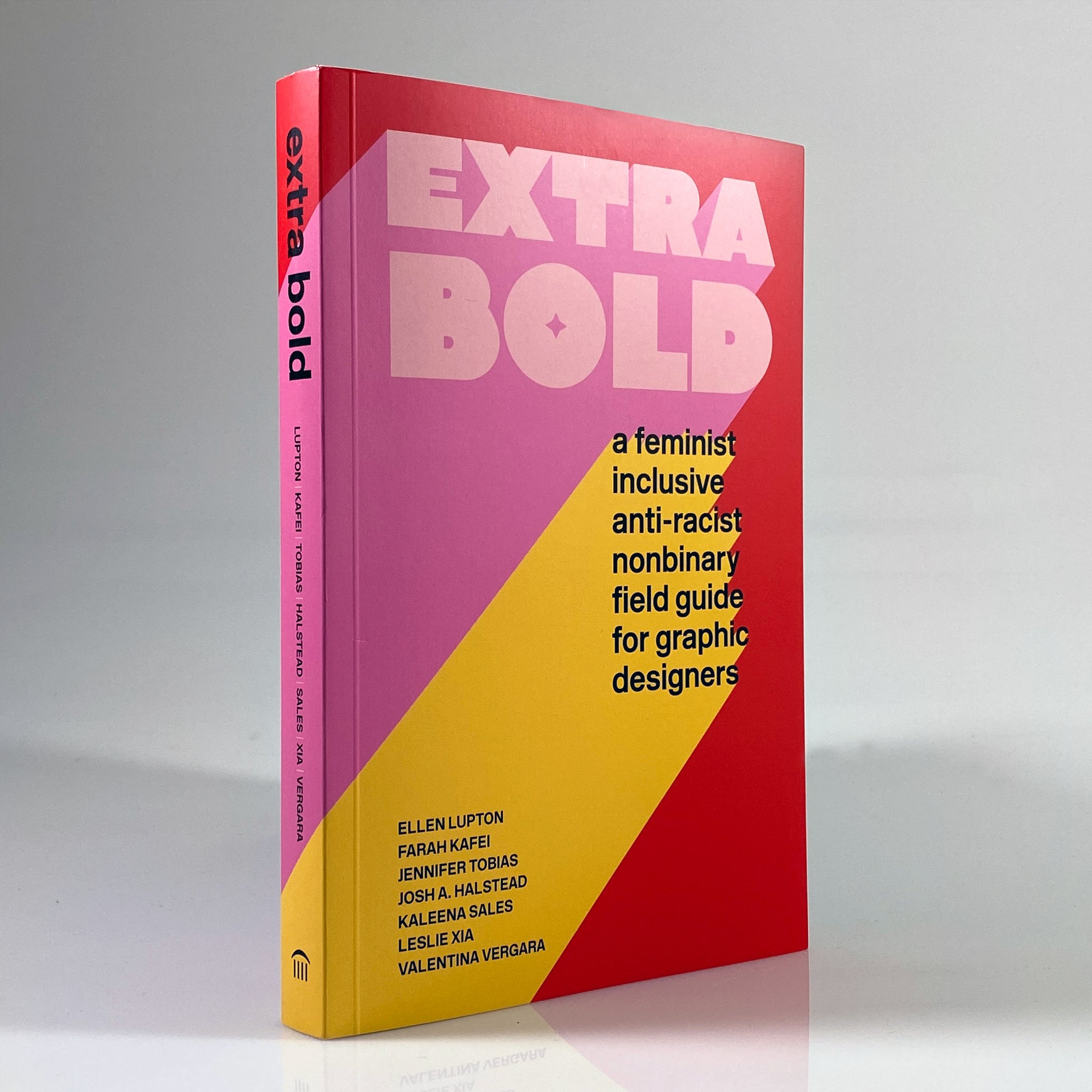The image features a prominently displayed book titled **"Extra Bold: A Feminist, Inclusive, Anti-Racist, Non-Binary Field Guide for Graphic Designers."** The book stands upright against a gray background and a light gray shelf. Its design is vibrant and captivating, characterized by a predominantly pink and yellow cover with an outer red band that wraps from the spine across the top and down the side diagonally to the right corner. The title "Extra Bold" is inscribed in large, bold pink letters at the top, accompanied by the subtitle in black letters below. The lower left corner lists the authors, including Ellen Lupton, Vera Caffey, Jennifer Tobias, Josh A. Halstead, and Leslie Zia. The spine of the book repeats the title "Extra Bold" and displays the authors' last names. A logo, presumably of the publishing company, appears at the lower part of the spine. The book casts a shadow, emphasizing its three-dimensional form, and is presented in a manner akin to a manufacturer's advertisement, suggesting a deliberate and proud display.